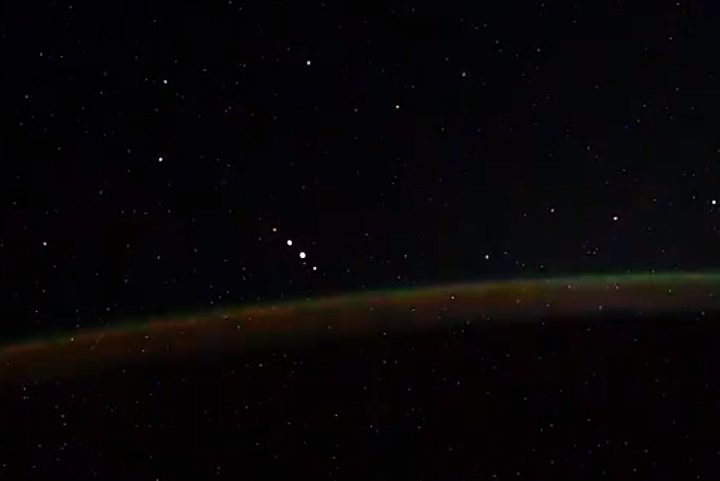This photograph presents a mesmerizing view of the night sky, likely a magnified image showcasing a star-studded expanse. The background is a deep, inky black dotted with variously-sized white and slightly colored spots, representing stars or planets. Prominently featured are three to four bright stars aligned in a diagonal row, suggesting a constellation, possibly Orion. The striking highlight of the image is a muted translucent band stretching horizontally across the center, exhibiting a gradient of greenish to reddish hues, reminiscent of a celestial phenomenon like the Milky Way or the Northern Lights. Beneath this band lies a dark, mass-like area with tinges of dark red, orange, and green, blending into the black of the sky, possibly depicting the edge of a planet or another astronomical feature. The image captivates with its intricate interplay of light and color, drawing viewers into the wonders of space.